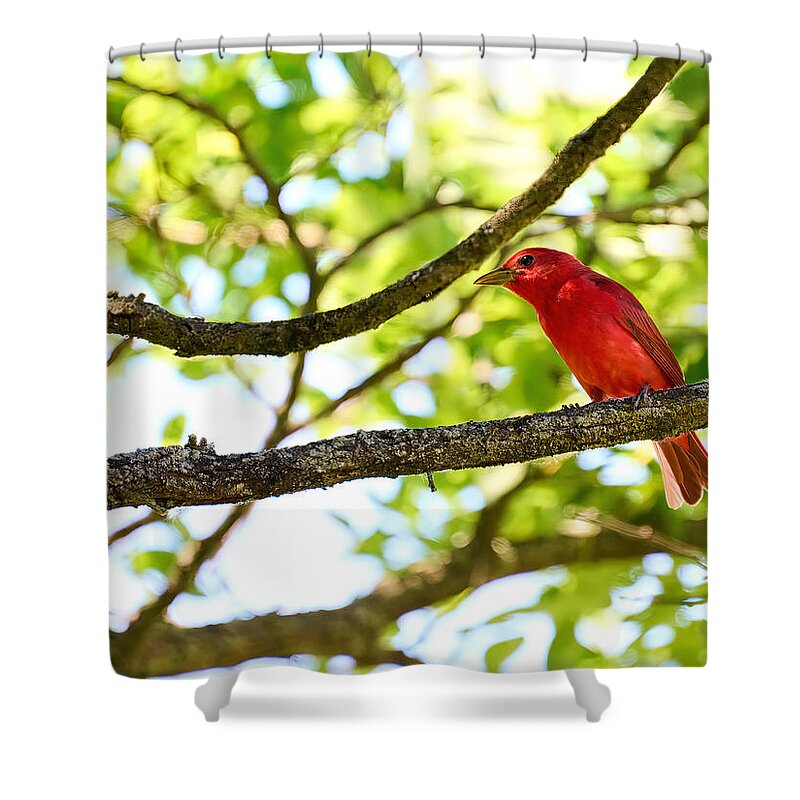The image showcases a vibrant red bird perched on brown, textured tree branches against a blurred background of blue sky and green leaves. The bird has bright red feathers with dark red accents, a yellow-brown beak, and shiny black eyes. It also features black stripes on its wings and some black markings on its tail. The entire scene is part of a high-quality shower curtain design, evident from the loops attaching it to a white horizontal bar at the top. The bottom of the curtain reveals the legs of a clawfoot tub, adding to the bathroom setting. The vivid colors in the image include shades of red, black, yellow, green, blue, and brown. There is no text or any branding visible, presenting the artwork as a professionally done piece intended to enhance the shower space.